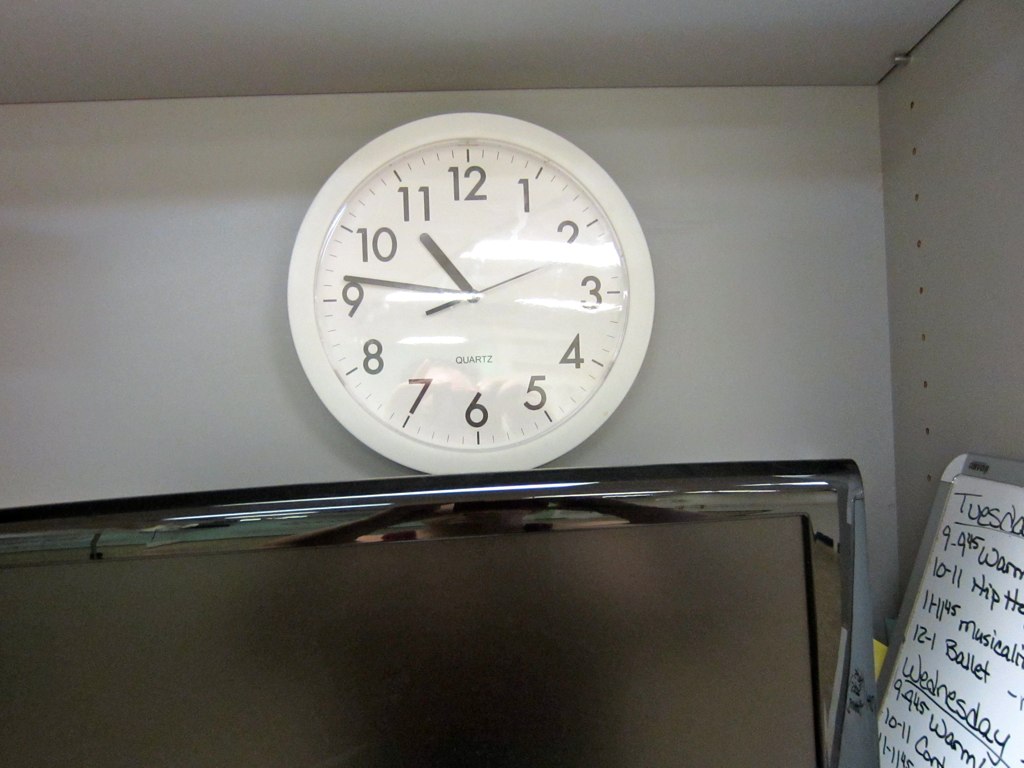This detailed photograph captures the interior of a cupboard where several items are neatly arranged. Dominating the lower third of the image is a black monitor with a glossy black trim that is currently turned off. Directly above the monitor, there is an analog clock featuring a white face encased in a white plastic housing. The clock displays the time as a little after a quarter to eleven, with the hour hand nearing 11, the minute hand slightly past the 9, and the second hand just past the 2. The clock face includes black numbers and minute markers, and reflects light prominently, revealing the word "Quartz" beneath the number six.

To the right-hand side, there is a whiteboard with a dark gray frame, positioned against the cupboard's side. The whiteboard lists a schedule that reads "Tuesday" followed by activities and times: "9 to 9:45 WAR," "10 to 11 [illegible]," "11 to 11:45 musician," and "12 to 1 ballet." For "Wednesday," it lists "9 to 9:45 warm up," alongside other partially obscured entries. The cupboard itself is gray and features small adjustable holes for shelving units visible along the right side, allowing for customization within the space. The overall lighting casts a grayish tone over the white surfaces, completing the organized and functional appearance of the cupboard's interior.